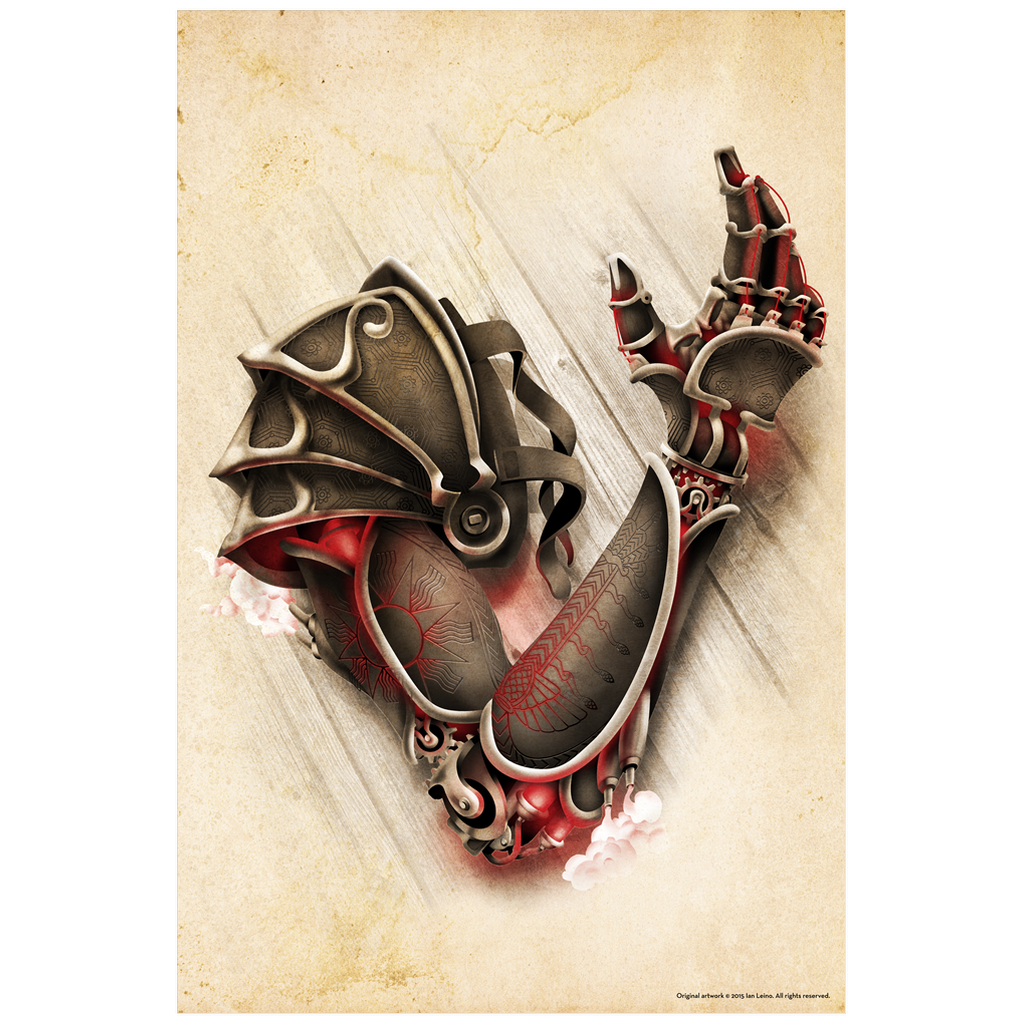The image showcases a detailed, digital artwork of an ape-like creature equipped with an ornate mechanical arm. The mechanical arm extends towards the right side of the frame and is intricately designed with jointed fingers and red tendons running through circuits. This robotic appendage features metal that extends from the hand, all the way up to the shoulder, adorned with a shoulder pad and straps for harnessing.

The arm, a blend of metal and leather, includes armor on the bicep, tricep, and forearm, each segment decorated with red glowing imprints and lined with vents that seem to emit steam. Red lights accentuate the mechanical aesthetics beneath the arm panels and within the hand itself. The shoulder armor consists of three segments, lined with metal and inlaid with brown leather.

Further details include a large armor plate over the forearm, the top of the hand, and the head of the creature. A round silver object encircles its eye, complemented by a cheek guard on the left side. Red tattoos extend from the hand's underside up to the arm. The ape-like figure appears to emerge from a light-colored hardwood surface, framed by cream edges.

In the bottom right corner, the artwork is credited with the text, "Original Artwork in 2005 by Lee Levine, all rights reserved." The overall style harmonizes digital artistry with a 3D-like rendering, contributing to its intricate and vivid depiction.